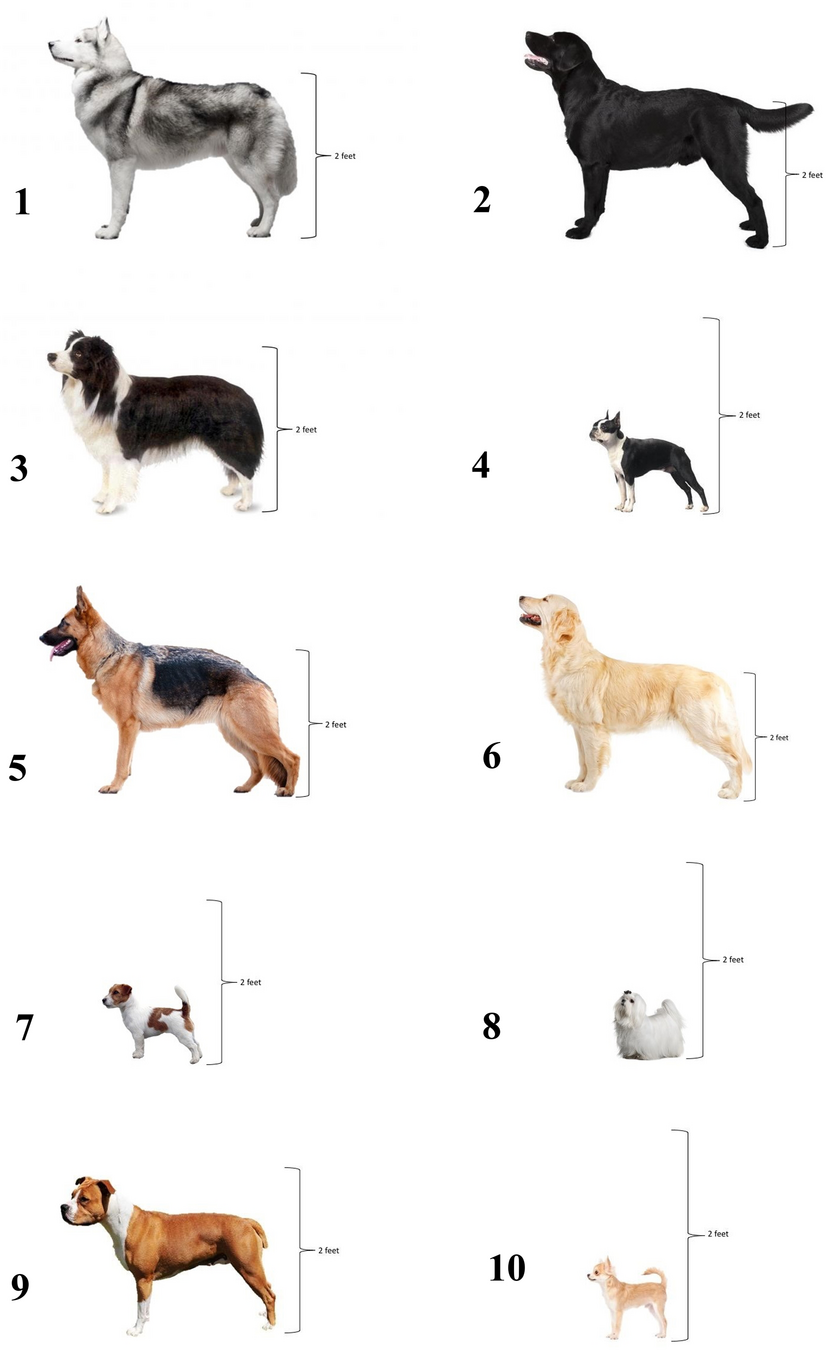This detailed image, suitable for a book or magazine, features 10 distinct dog breeds, all labeled and arranged in two columns of five rows each, for a total of ten profiles. Each dog is presented in a left-facing side view, colored to depict their natural appearances. The breeds, positioned from largest to smallest, include an Alaskan Husky at number 1, a black Labrador Retriever at number 2, a Border Collie at number 3, a Bulldog at number 4, a German Shepherd at number 5, a Golden Retriever at number 6, a Jack Russell Terrier at number 7, a Pekingese at number 8, a Bulldog or Boxer at number 9, and a Chihuahua at number 10. 

A vertical scale marked with a "2 feet" indicator is present to the right of each dog, allowing viewers to compare the relative sizes of the breeds. This scale reveals that while each dog's height is shown up to 2 feet, their true heights vary significantly. For instance, the Alaskan Husky and Labrador Retriever approximate the 2-feet mark, while the Border Collie is just about 2 feet tall and the Bulldog is slightly shorter. This detailed comparison not only contrasts heights but gives readers a clear visual reference of each breed's stature, making it a valuable resource for understanding the size variations among popular dog breeds.